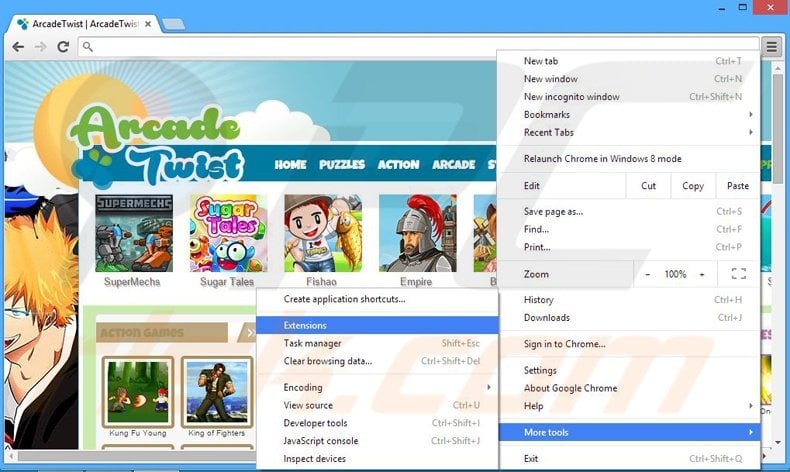The image titled "Arcade Twist" showcases a vibrant assortment of gaming icons, each representing different genres ready to be played. Highlighted categories include Home, Puzzle, Action, and Arcade, creating a dynamic interface for users. Among the notable games displayed are "Super Mecha" and "Super Tails" featuring playful, animated characters including a quirky, wide-eyed animal. Another game, "Fishio," depicts a red-headed boy proudly holding up a fish, adding to the image's lively atmosphere. Buttons for "Empire" and two Kung Fu themed games, "Kung Fu Gang" and "Kung Fu Fighters," are also visible.

In the foreground, a portion of a website interface is shown, where the user is navigating through the "More Tools" menu. Adjacent to it, an extension tab is opened, highlighting the user's intention to modify or enhance their gaming experience with possible extensions. The scene captures a moment where the user is in the process of adding these extensions to optimize their interaction with the arcade games, aiming for a tailored and enriched gaming session.